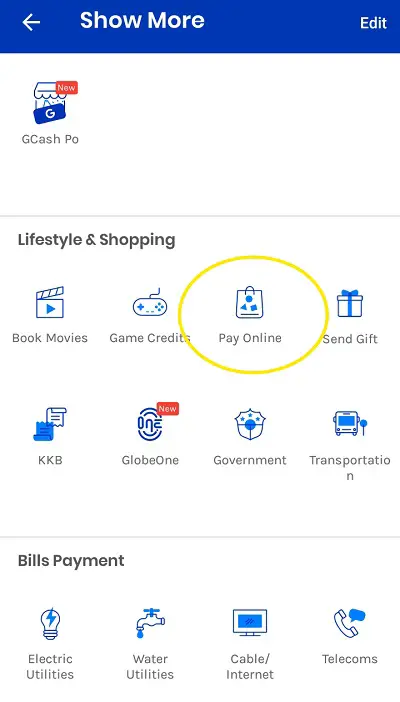The image showcases a digital interface with multiple features and options presented in a well-organized layout. On the left side, there is an arrow pointing to the left, indicating a navigation option. The interface includes categories like "GCash Pro Lifestyle" and "Shopping." It also highlights various service sections such as "Books and Movies," "Game Credits," and "Pay Online," with the "Pay Online" option circled for emphasis.

There is a "Send Gift KKB" feature and a "Globe One" section, the latter styled with a capital 'G' and capital 'O' as one word. At the top, a red rectangle with the word "New" in white text draws attention to newly added features. It indicates options for paying government fees, transportation bills, electric utilities, water utilities, cable, internet, and telecommunications services.

A second red rectangle also labeled "New" in white text appears at the very top of the image. All these elements are likely part of a comprehensive mobile app interface designed to facilitate various financial transactions and services seamlessly.